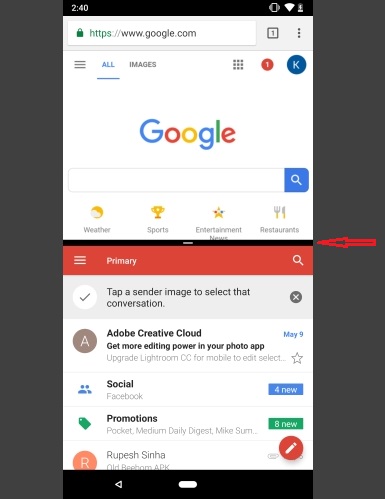The image showcases a standard Google search page. At the top, the URL bar displays "HTTPS" in green, indicating a secure connection, followed by "www.google.com." Below the URL, the iconic, colorful Google logo is prominently featured, consisting of a blue 'G', red 'O', yellow 'O', blue 'G', green 'L', and red 'E'.

Directly beneath the logo is the primary search bar. Above this, the "All" tab is highlighted in blue, suggesting that it is the current selected option. If an alternative category, like "Images," were clicked, it would lead to image search results.

Below the search bar, there are category links for "Weather," "Sports," "Entertainment," and "Restaurants." Following these links, there exists a prominent red rectangle labeled with the "Primary" tab, accompanied by an additional search function. 

Highlighted in a gray rectangle is a message indicating that the option to "Tap a sender image to select that conversation" has been checked.

Further down, an advertisement for Adobe Creative Cloud offers an upgrade to Lightroom CC for mobile with more editing power. Following the ad, there is a notification from Facebook indicating four new messages. 

In the "Promotions" section, there are messages from various sources, including "Pocket," "Medium Daily Digest," and a partially displayed message from "Mike Sum" with eight new notifications. 

At the bottom, there is a message from Rupesh Sinha regarding "Old Reborn APK." Nearby, a clickable red circle allows users to compose new information. The entire layout is meticulously structured, designed to facilitate easy navigation and user interaction.